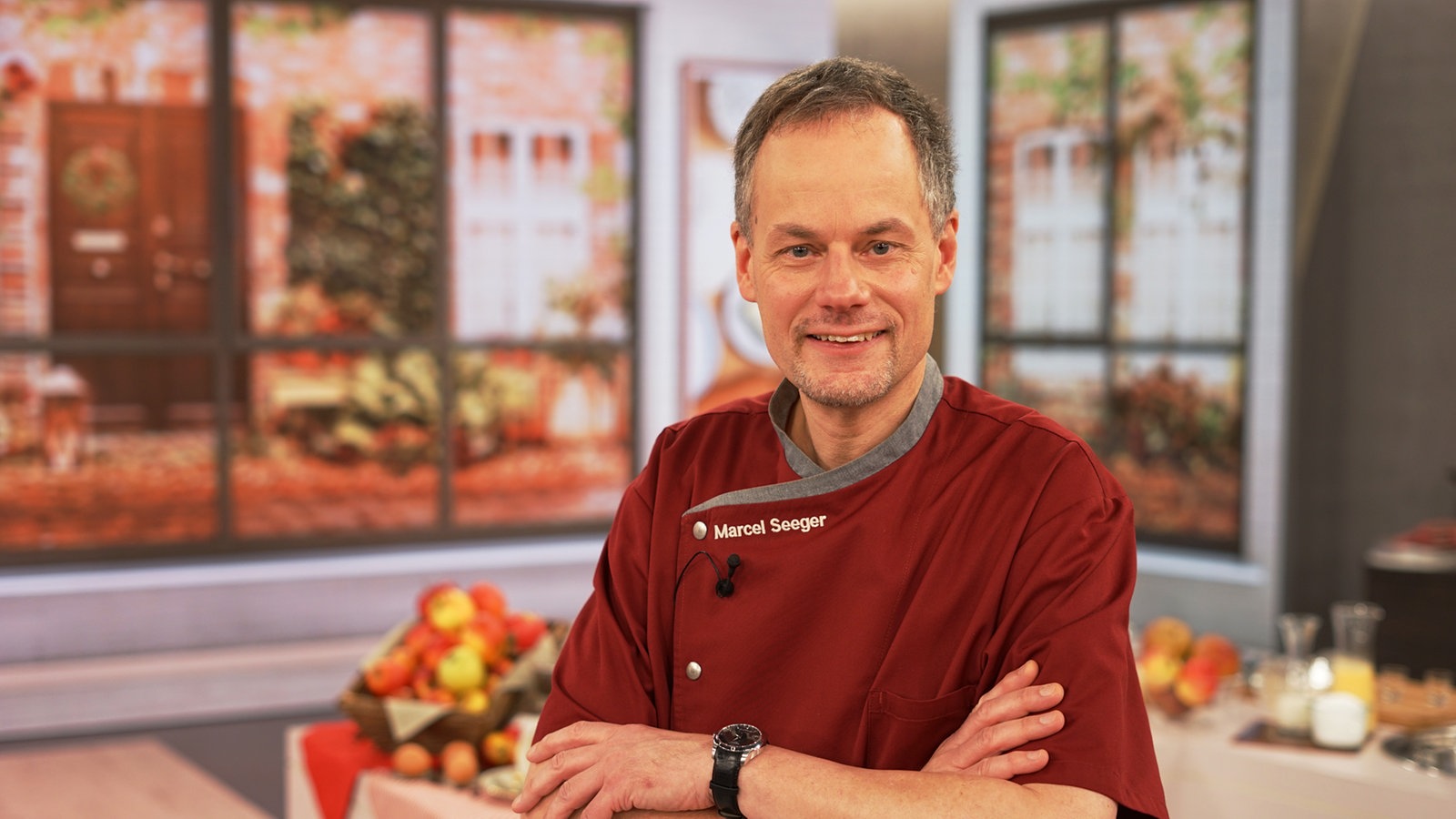This detailed photograph captures an older, slender man named Marcel Seeger standing in what appears to be a studio setting, likely for a cooking show. Marcel, wearing a burgundy chef's shirt with gray trim around the collar, has a small microphone clipped to his shirt and a black watch on his left wrist. His arms are crossed, and he sports a friendly smile, with dark hair and a hint of stubble on his face. Behind him is a table laden with an assortment of fruits, primarily apples, and other food items, though the exact details are slightly out of focus. The backdrop features a faux window scene that gives the impression of an autumnal landscape, including a view of another house with visible windows and a front door, further suggesting an outdoor courtyard setting.